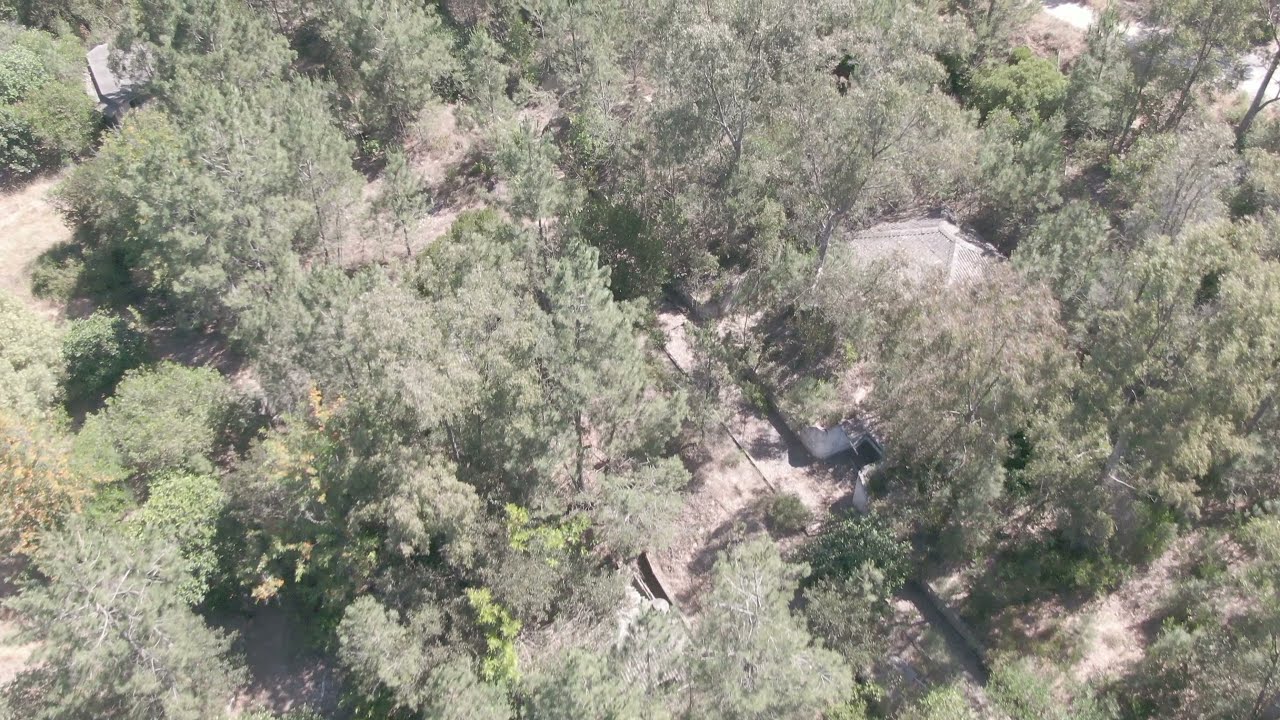This aerial image captures a densely wooded area during summertime, where the sunlight filters through the canopy, revealing a spectrum of green hues. The scene is predominantly marked by a variety of trees, including pine trees and others with full green leaves, showcasing the natural density of the forest. Interspersed among the greenery are small patches of tan-colored ground, hinting at areas of dirt and possibly dead grass.

Nestled within this natural expanse are a few structures that blend into their surroundings. In the upper left-hand corner, a small building peeks out from between the trees, while a slightly larger building can be glimpsed in the center right-hand side. Both structures appear to have gray roofs. Additionally, there is a faintly visible road or trail running diagonally across the image, partially obscured by the forest canopy, connecting these hidden homes. 

The colors in the image range from various shades of green to beige, gray, and brown, enhancing the sense of a rural and secluded setting. The overall atmosphere indicates a location far from urban environments, where nature predominates and human presence is subtle yet integrated into the landscape.